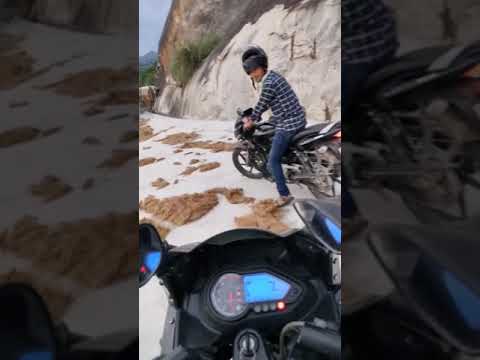In this vertical cell phone style photograph, we see a dynamic first-person perspective from someone on a motorcycle, likely captured using a GoPro. The foreground features the visible front of the photographer's motorcycle, including a speedometer and additional instrument details, with partially visible mirrors on both sides. Directly ahead, another man on a motorcycle looks back towards the camera. He stands out in a dark, checkered plaid shirt with white stripes, blue jeans, and sandals. Notably, the man is sporting a distinct Russian-style fur hat rather than a helmet, contrasting with the overall rugged surroundings.

The setting is a rocky area with a curved rock surface leading up to a sheer rock wall. Brown patches of vegetation are scattered across the ground, hinting at a dry, sand-like terrain. The background sky is a muted gray, suggesting an overcast day. The entire scene is framed by an enlarged, faded version of the same image, providing a sense of depth and focus on the central action: the interaction between the motorcyclists amidst this rocky, vegetated landscape.